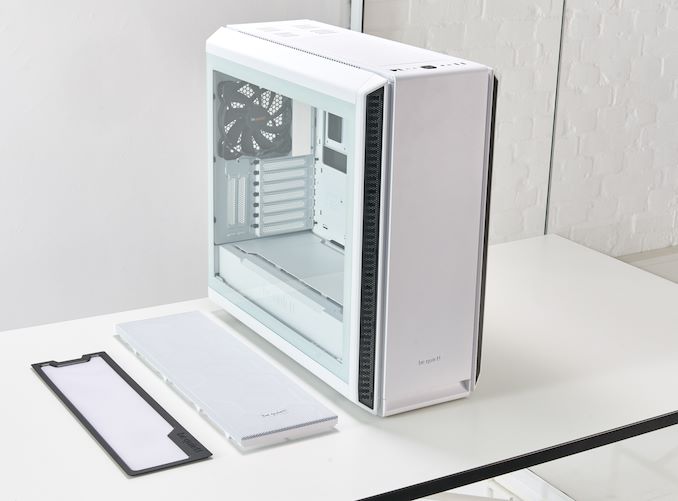The image depicts an empty white computer tower case, centrally positioned on a white table with black edging. The side panel of the case is open, revealing a completely hollow interior, devoid of any computer components. The exposed interior shows several metal slots and fasteners intended for future installation of hardware, as well as a black vent on each side designed for airflow and cooling. The case's exterior is predominantly white, with black accents along the sides. On the table in front of the case lay the side panels: one being white with a black trim, and the other appearing mostly gray. In the background, against a backdrop of white walls, an indentation is noticeable on the right side, while the left wall remains smooth. There's some writing visible on both the bottom and top of the case, though the exact text is unclear. The scene is very clean, with a minimalist color palette of whites, blacks, and grays, evoking a ready-to-build aesthetic for the computer tower.